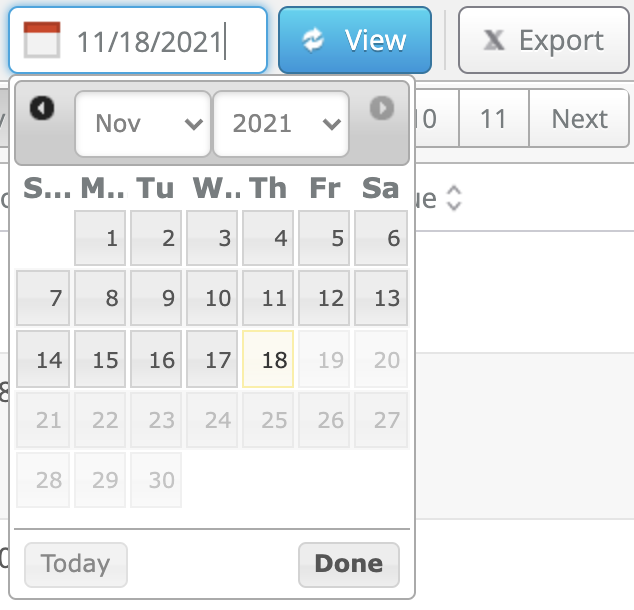In the image, a screenshot of a digital calendar is displayed prominently. Toward the upper left-hand corner, there is a box with a calendar icon to its left, containing the date "11-18-2021." An interactive calendar pop-up is visible, indicating the selected month as "November 2021." This calendar adheres to a Sunday-to-Saturday format, with November 1st starting on a Monday and November 30th ending on a Tuesday.

At the bottom of the calendar, there are two buttons: the "Today" button on the left and the "Done" button on the right. In the upper right-hand corner of the screenshot, an "Export" button is visible. Beneath the calendar pop-up, there are sections partially obscured by the calendar. On the right side, buttons labeled "10," "11," and a "Next" button are visible. Further down, another section's end can be seen with a letter "E" and adjacent up and down arrow buttons. Three additional sections are present but are completely covered by the pop-up calendar, leaving their text unreadable.